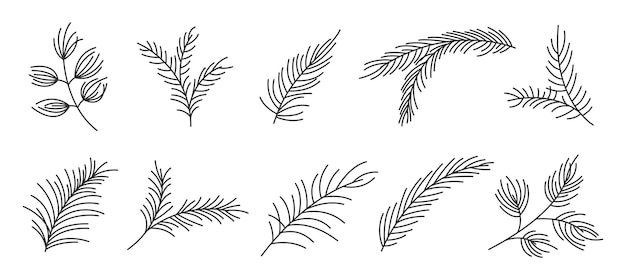The image displays a collection of black line drawings of various leaves and twigs, set against a stark white background. There are ten individual illustrations, organized in two horizontal rows with five designs in each row. The drawings are simple yet detailed, showcasing different classifications of leaf and twig structures, primarily focusing on needle-like leaves. The stems are drawn on the left, with leaves depicted in clusters or branches extending outward. Some illustrations portray single branches with evenly spaced needles, while others show more complex structures like curly needles or branches that split in the middle. The image is devoid of any text or numbers, enhancing the clarity and focus on the detailed botanical line art, rendered exclusively in black on a bright, illuminated white setting.